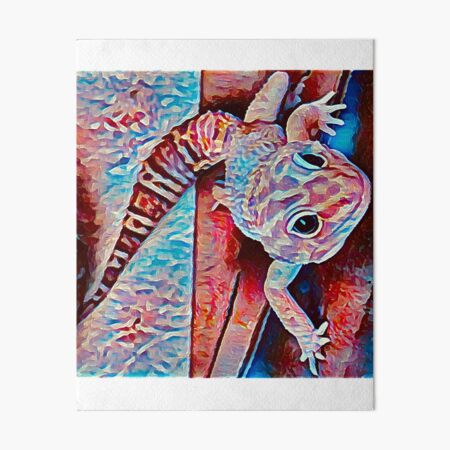This painting depicts a vibrant reptile, potentially a lizard or gecko, positioned as if it is climbing a wall. The image itself is contained within a small, square frame approximately three inches high and wide, set against a light gray, almost white background. The inner rectangle, around two inches high by one and a half inches wide, features thin white headers and footers at the top and bottom.

Inside this frame, the reptile is situated on the right-hand side, with its head turned to the right and its body trailing beneath, extending its long, striped tail towards the left. The tail showcases a pattern of maroon, red, and light white stripes. The background is split into two contrasting sides: the left half tinged with blues and touches of red, and the right half dominated by reds with hints of blue.

The reptile itself is a colorful spectacle with blue eyes and striking blue eyelids. Its face is adorned with red and yellow stripes, while its back displays shades of blue and yellow. The limbs of this four-fingered creature add to its detailed depiction. The overall coloration of the reptile includes blue, white, brown, red, black, and gray, making it a vivid and intricate subject within the small, meticulously divided painting.